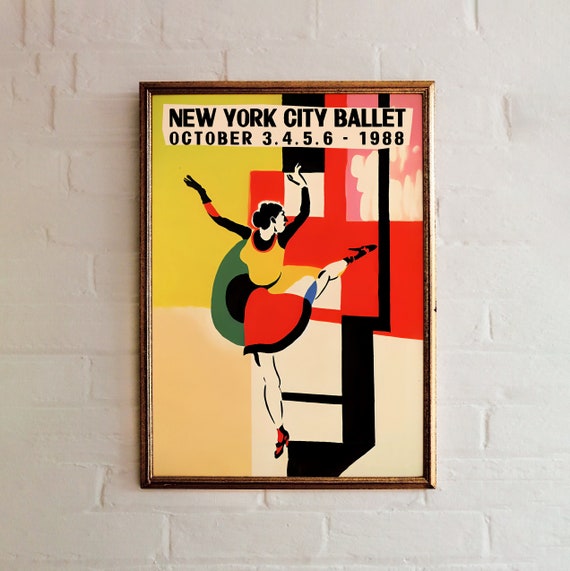This is a detailed description of a framed poster hanging on a white brick wall. The frame is made of gold metal. The poster advertises the New York City Ballet with the text "New York City Ballet, October 3, 4, 5, 6, 1988" prominently displayed in bold black letters within a cream-colored rectangle at the top. The artwork is abstract, featuring a ballet dancer at its center, gracefully posed with her leg kicked backwards, head turned to the side, and hands lifted in the air. The background is divided into sections of varying colors and geometric shapes: the top left is yellow, the bottom left is a mix of tan and darker green, the bottom right is monotone black and white, and the top right combines red, black, white, blue, and pink. The composition of these colorful, modern blocks adds a dynamic and artistic flair to the overall image.